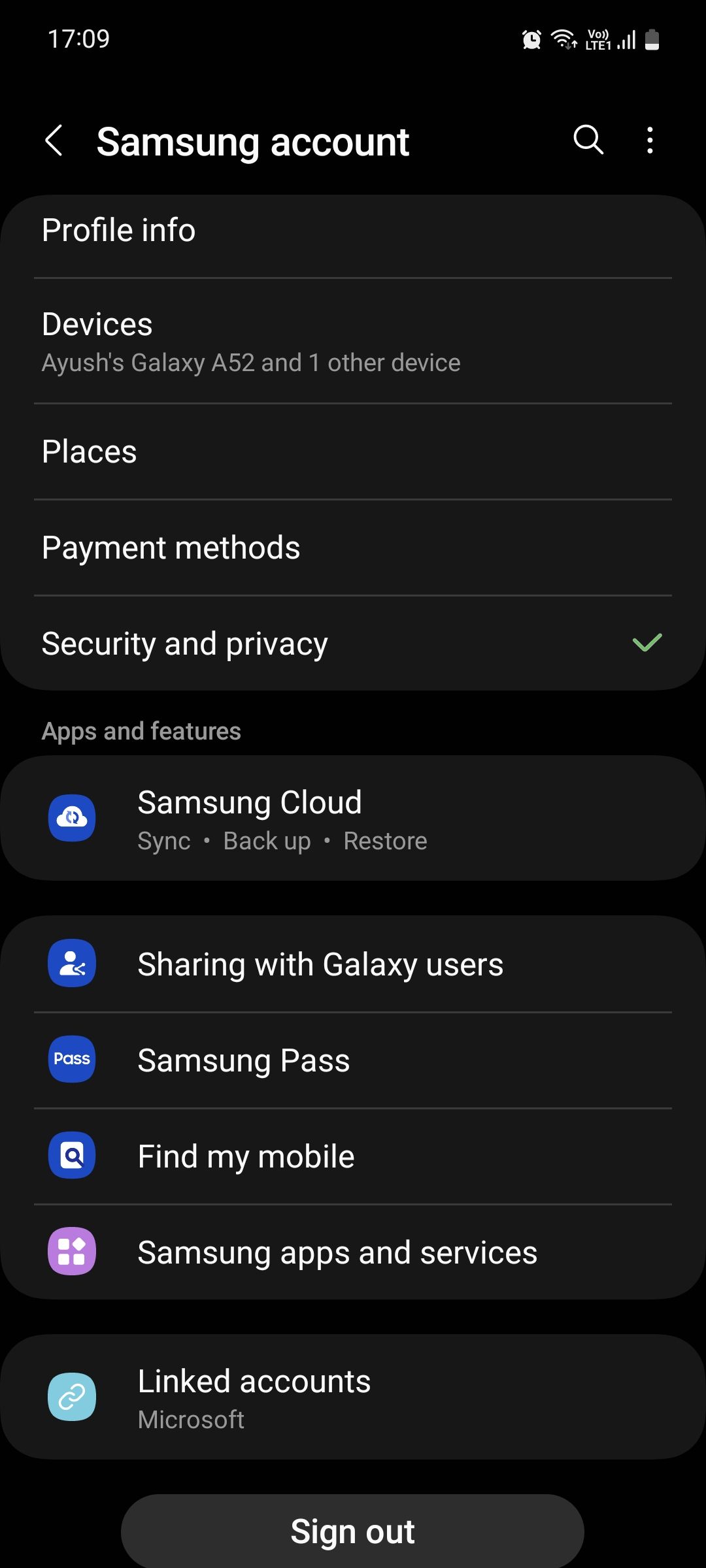A detailed caption for the provided image could be:

"This screenshot captures the settings interface of an Android mobile phone, specifically a Samsung device as indicated by the 'Samsung' branding visible on the screen. The phone's status bar, showing a battery percentage icon in the top right corner, confirms it's a mobile device. The interface is displaying the Samsung account management section, which is set to dark mode, as evidenced by the dark background and contrasting white text. The visible settings include options to manage profile information, devices (listing 'AYUSH's Galaxy A52' and one other device), places, payment methods, and security and privacy settings. Also notable are options for Samsung Cloud, sharing features with other Galaxy users, Samsung Pass, Find My Mobile, Samsung Apps and Services, and linked accounts. The user interface features a back button at the bottom left and a magnifying glass search icon at the top right, along with a three-dot menu for additional options. A prominent 'Sign Out' button is also displayed, suggesting it provides a quick way to log out of the Samsung account. The current time is displayed as 5:10 pm."